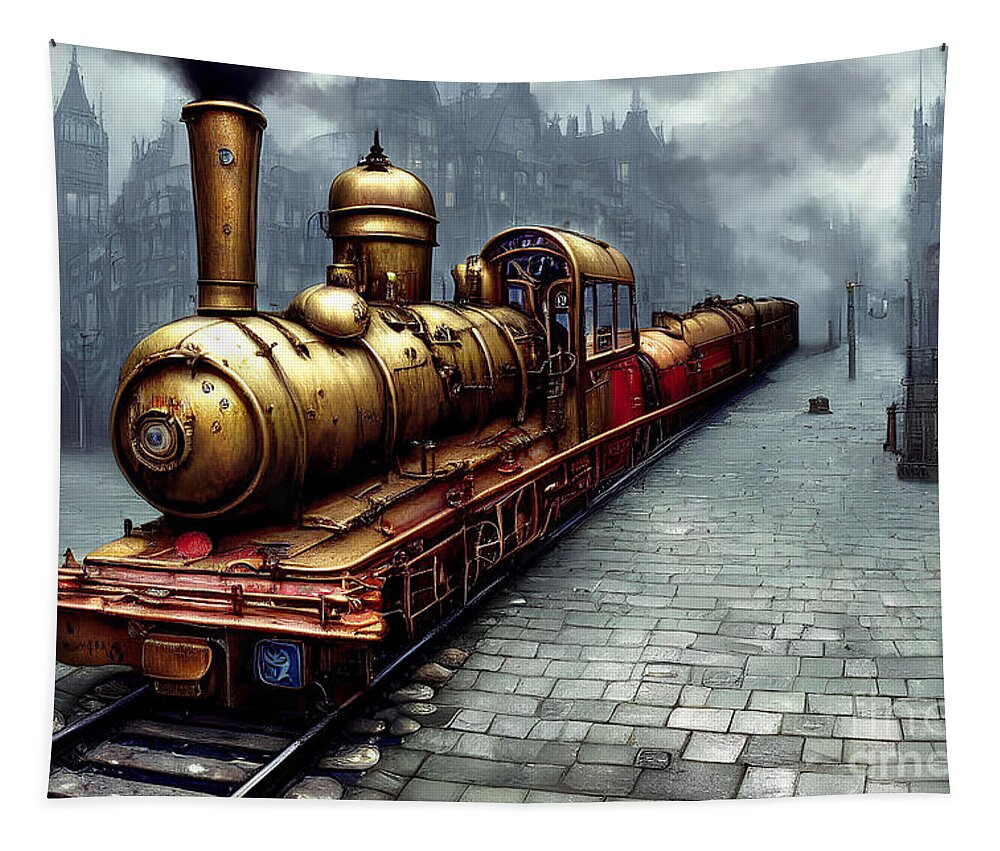The image depicts a vintage steam locomotive, seemingly from the late 18th or early 19th century, rendered in a detailed, painterly style that evokes historical artwork. The locomotive, painted in a light brown or copper hue with brass and steel elements, emits dark smoke from its stack, suggesting active operation. It features a flat bed and intricate piping along its boiler section. The front coupling is visible, though the wheels are obscured by shadow. Behind the engine, there are three or four short train cars, unlike typical freight cars, possibly used for specialized cargo or passengers. The train runs on steel tracks flanked by a cobblestone path, which appears grayish and extends into the distance, framing the scene. The background is enveloped in fog and darkness, dominated by a towering structure that could be a mansion or hotel, distinguished by its multiple stories and numerous windows. The sky overhead is cloudy and grey, contributing to the overall somber and historical atmosphere of the setting. The entire image is presented as if printed on fabric, with visible nails at the top corners and a slight slope, adding to the impression of an antique, possibly European, landscape.